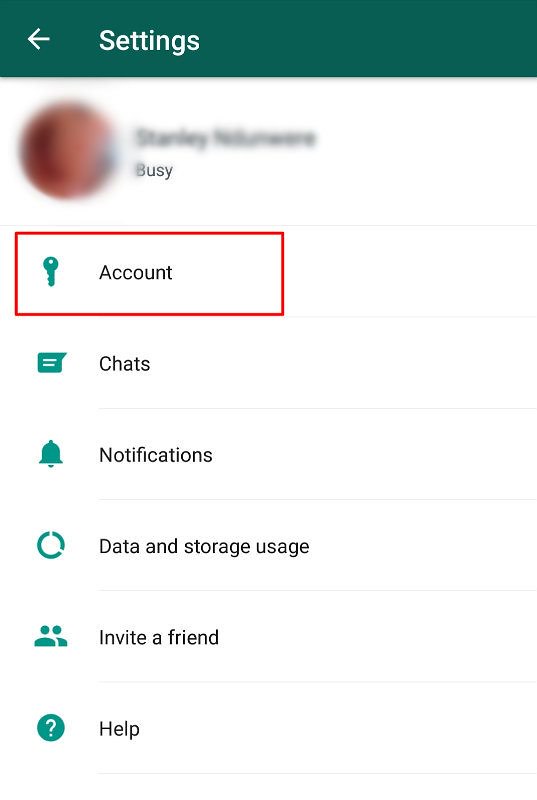A detailed image caption is as follows:

This image shows a computer screen displaying a user interface of a program. Prominently featured is a blurred-out profile, with an icon that appears to depict a person, accompanied by a name. Although the name is partially obscured, the first name appears to be "Stanley," with an indistinct, lengthy last name. At the top of the screen is a green box with an arrow pointing left, containing the word "Settings" in white text. Beneath the blurred name, the status is marked as "Busy." Below this status, there is a red box highlighting the word "Account," which is accompanied by a key icon, symbolizing security or login information.

Further down, there is a section labeled "Chats," featuring an icon resembling a speech bubble or text message. Next is the "Notifications" section, indicated by a bell icon. There is also an option labeled "Data and Storage Usage" next to a circular icon. Below, the interface offers an "Invite a Friend" feature, depicted with an icon of two stylized figures, one slightly larger than the other, representing users. At the very bottom of the screen, a green circle encloses a question mark next to the word "Help," indicating assistance or support options. The interface seems designed to facilitate access to various settings and options, such as account management, chats, notifications, and data usage for the user, whose specifics are intentionally blurred for privacy.